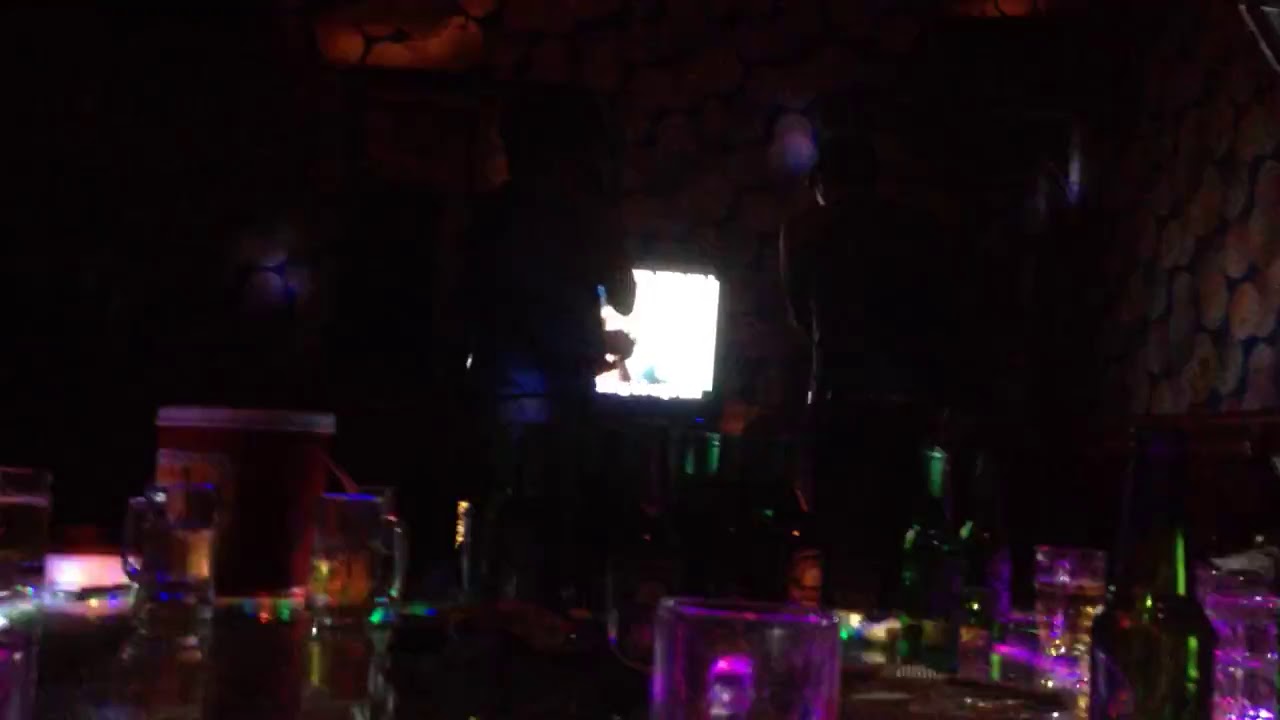The image depicts a dimly lit, indoor setting that closely resembles a bar, characterized by its dark, cavernous ambiance. In the center of the composition, there is a bright white square that could be a TV screen or a window letting in natural light. To the left of this bright area, there is a shadowy figure, possibly a person, with their elbow faintly visible.

The background features walls that are designed to mimic tan stone, enhancing the rustic, bar-like atmosphere. On the countertop in the foreground, there are several beer mugs and bottles. Notably, there are green and amber-colored glass jars, along with at least one full beer mug, another half-full, and an empty one closest to the camera. Some glass items appear to be illuminated with hues of pink and purple, adding subtle, colorful accents to the otherwise dark space.

No other people are visible in the image, suggesting it might be a bar after hours or during a quiet moment. The combination of the stone walls, varied lighting, and assortment of drinks contribute to the overall impression of a secluded, cozy bar environment.